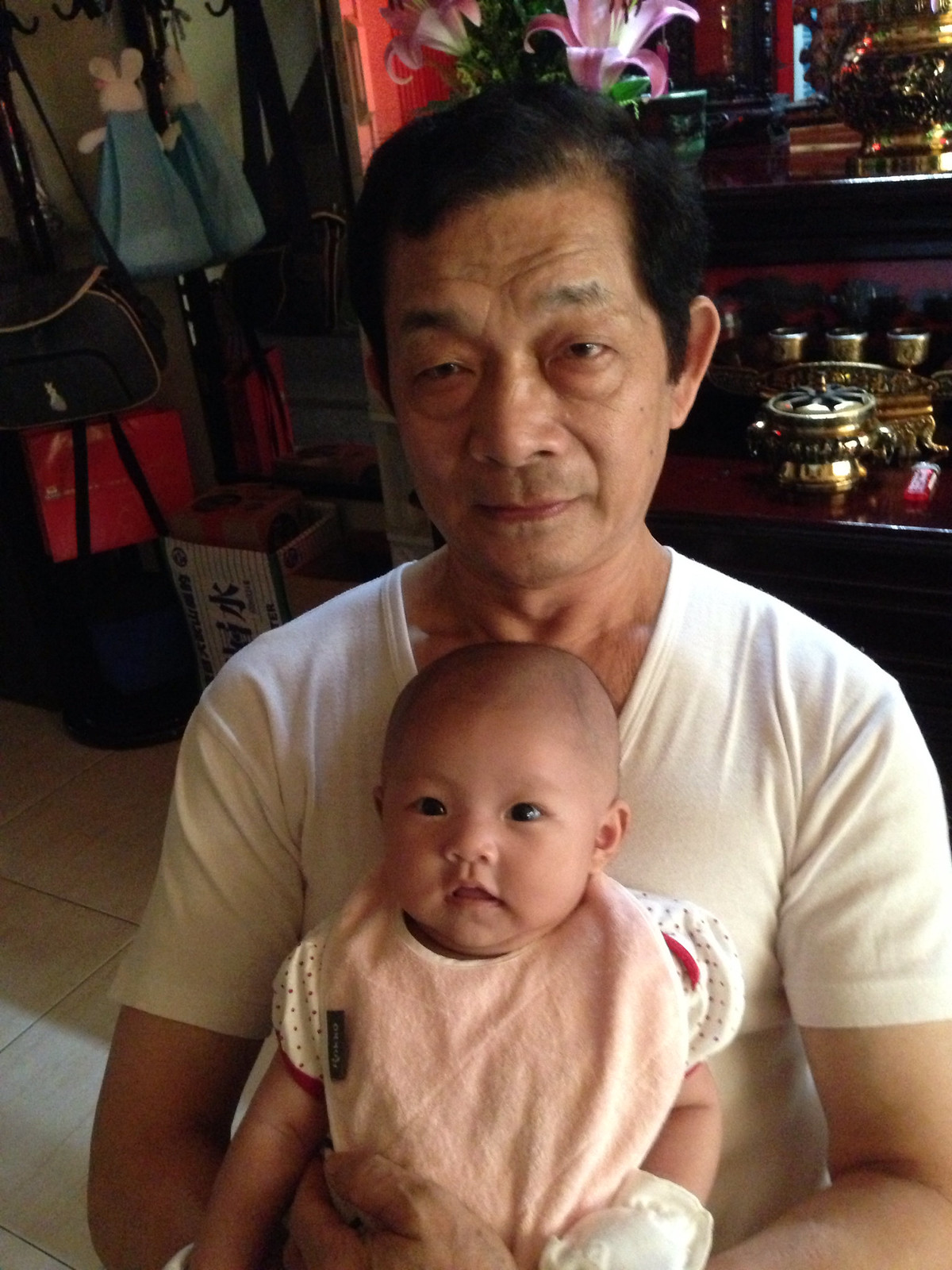In the photograph, an older man, possibly in his 60s or early 70s and of Asian or South Pacific descent, is sitting with a young child on his lap, likely his granddaughter. The man has dark black hair and is dressed in a plain white v-neck t-shirt. The child, who appears to be a baby girl, is wearing a light pink bib over a white onesie adorned with black polka dots. The man's arms gently encircle the baby’s midsection as she gazes forward, expressionless.

The setting appears to be indoors, potentially a boutique or store. In the background, there is a mix of objects that add to the scene's detail: an Easter Bunny decoration, some purses and lunch bags, a wooden cabinet filled with brass pots and small trinket boxes, as well as a display of pink and white tiger lilies with green leaves. Additionally, there is a red cardboard box and what could be interpreted as a golf club bag. The photo captures a moment that blends familial warmth with an eclectic assortment of background items, predominantly featuring colors like white, pink, brown, and red.